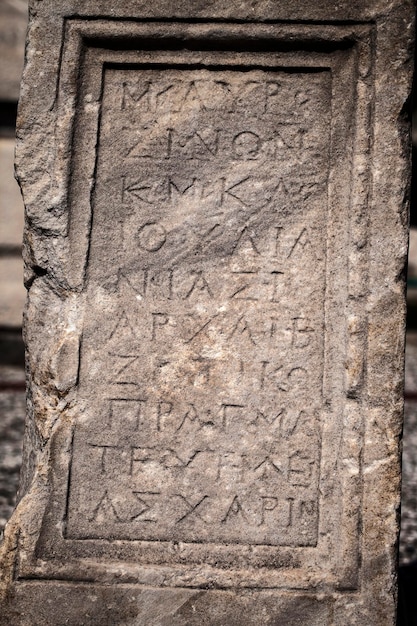The image depicts a very old, ancient-looking rectangular stone tablet that is taller than it is wide. The edges of the tablet are significantly damaged, with the entire left-hand side broken and chipped away, resulting in no clean or intact borders. A large chunk of stone is missing from the edge, and the remaining portions show signs of heavy wear and aging. The surface of the stone is predominantly gray, but it features areas of lighter gray, brown, and beige, particularly dirty and almost blackened in the lower portion and the top right corner, likely due to accumulated dirt or grime over time.

The tablet has an ornate carved border and frame in the middle, within which lies a flattened surface inscribed with indecipherable writings. The inscribed letters resemble those of the Greek alphabet, displaying characters such as omega (Ω), alpha (Α), and epsilon (Ε), although some might argue they could also be Roman letters due to their appearance. The carvings stretch from the top to the bottom of the stone slab, likely created using a chisel. Despite attempts to identify the specific letters, they remain largely unrecognizable, contributing to the mysterious and ancient aura of the tablet.